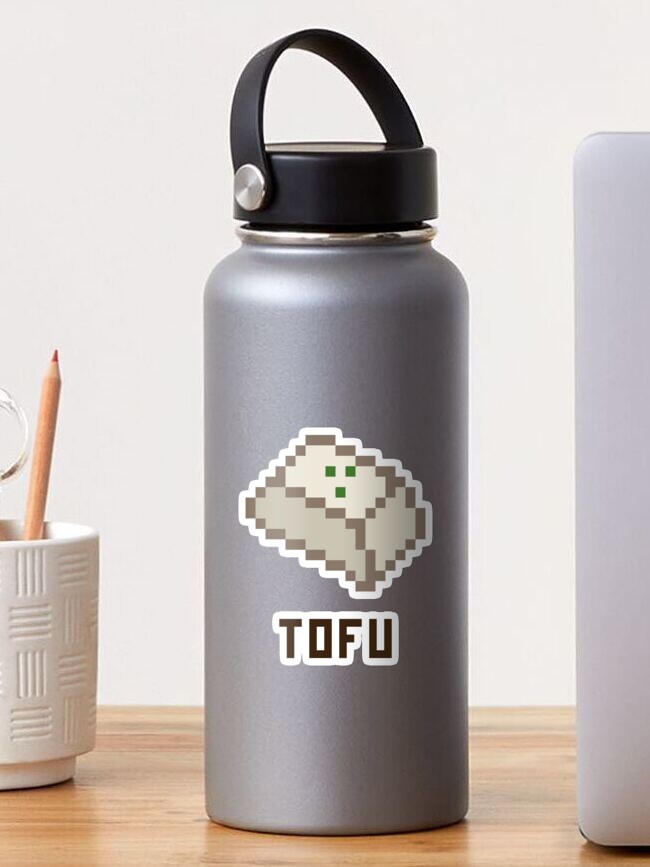The image features a close-up of a gray metal hydro flask prominently placed at the center of a wooden brown table. The hydro flask is equipped with a black screw-on plastic lid featuring a small handle loop, which is only large enough to fit a hand through. The hydro flask itself is adorned with two stickers in the middle: one near the bottom half spelling "tofu" in medium-sized letters, and directly above it, a pixelated cartoon image of tofu. This cartoon tofu is light green in color, with green eyes and a green mouth, all represented by pixel squares, accompanied by three small garnish bits. To the left of the hydro flask is a modern pencil holder, partially visible, containing a colored pencil with its point sticking up, and possibly the handle of a pair of scissors. On the right side of the flask is the slightly cut-off edge of an open MacBook laptop. The background is blank, focusing attention on the objects resting on the table.